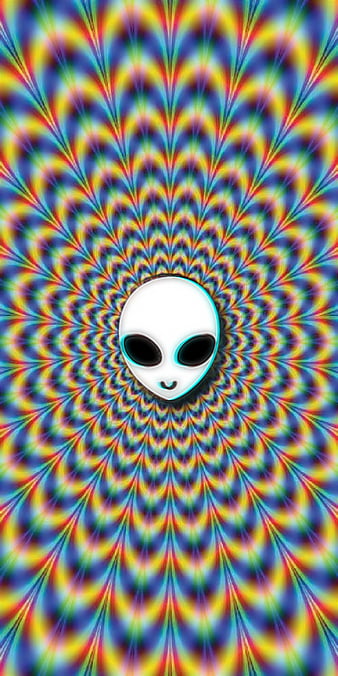The vertical rectangular image features a central alien face, depicted with a stereotypical white, egg-shaped head, large black eyes, and a small, upward-curving smile. Surrounding the alien head is a holographic, psychedelic background that appears to move and pulsate with the viewer's perspective. The background comprises approximately 20-25 concentric, feather-like arcs that radiate outward from the alien face, starting small and growing larger towards the edges of the rectangle. These multicolored, squiggly lines, reminiscent of turkey tail feathers, give a disturbing, wavy effect that intensifies the illusion of motion. The arcs display a rainbow-like spectrum of colors, enhancing the image's dynamic and psychedelic nature.